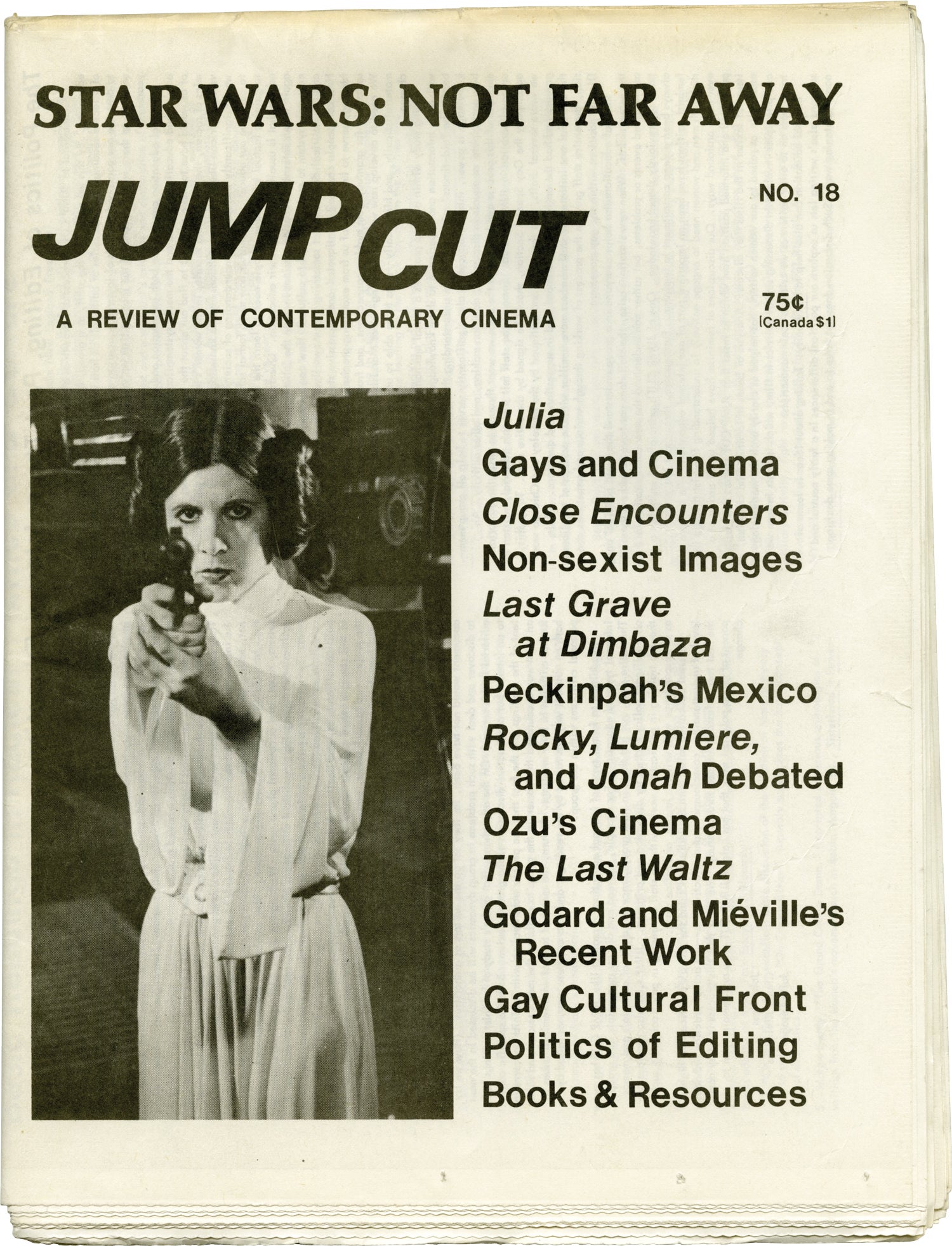This is a black and white scan of what appears to be an old magazine or newspaper dedicated to cinema, focusing on its front cover. The issue is titled "Star Wars Not Far Away" and is part of a series called "Jump Cut: A Review of Contemporary Cinema," specifically issue number 18. The price is marked as 75 cents, or one dollar in Canada. Prominently featured on the left side of the page is a black and white photograph of Princess Leia, portrayed by Carrie Fisher, from the original Star Wars film. She's holding a gun aimed directly at the viewer. To the right of this image is a column of text listing various articles and topics covered in this issue, including: "Julia," "Gays in Cinema," "Close Encounters," "Non-Sexist Images," "Last Grave at Dimbaza," "Peckinpah's Mexico," "Rocky," "Lumière and Jonah Debated," "Ozu's Cinema," "The Last Waltz," "Godard and Melville's Recent Work," "Gay Cultural Front," "Politics of Editing," and "Books and Resources." The entire page is presented in a classic black and white format, suggesting its vintage nature.